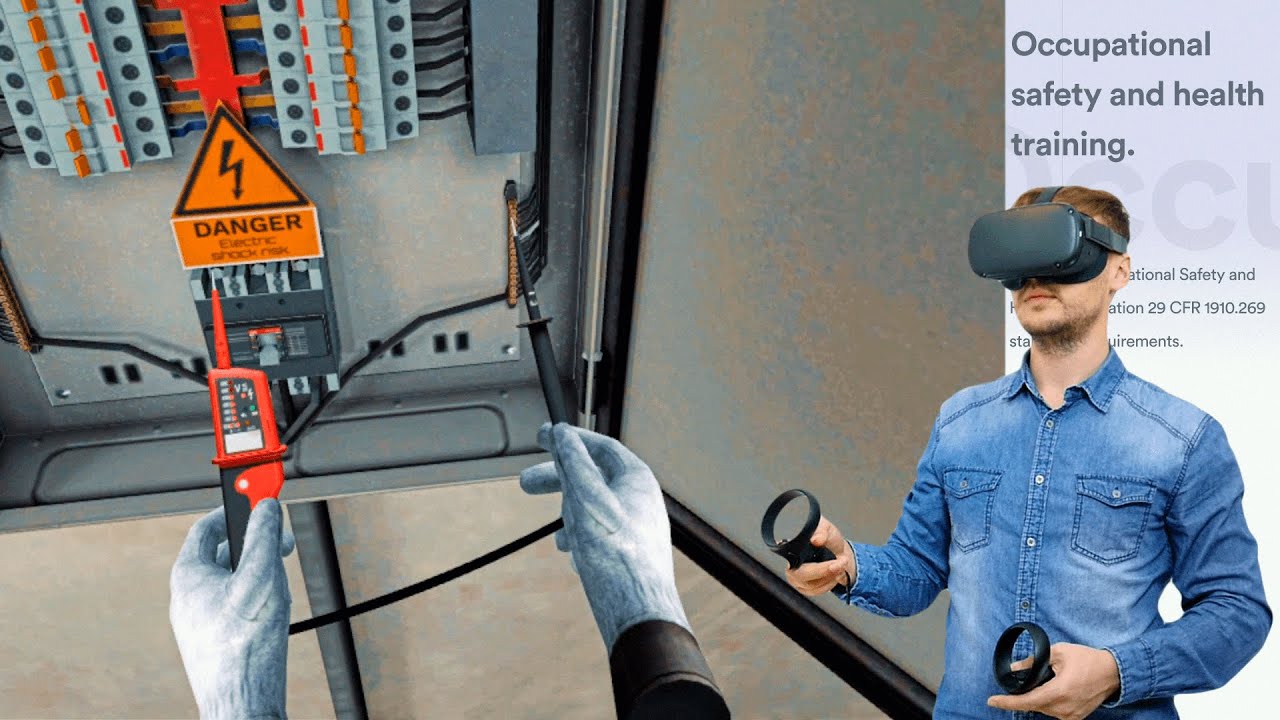A white male in his 20s or 30s, wearing a denim button-up shirt, is depicted on the right-hand side of the image, immersed in Occupational Safety and Health Training through a black MetaQuest VR headset and controllers. The VR simulation shows his virtual hands, donned in gloves, carefully handling a voltage meter with two prongs at a fuse box filled with orange fuse switches. One prong is grounded on a hinge while the other checks the fuses. Prominently displayed on the virtual fuse box is a yellow sign reading "Danger: Electric Shock Risk." The man appears superimposed over a detailed scene of electrical safety training, emphasizing the educational content of the simulation. This overlay gives a comprehensive view of both the digital environment and the hands-on training application.